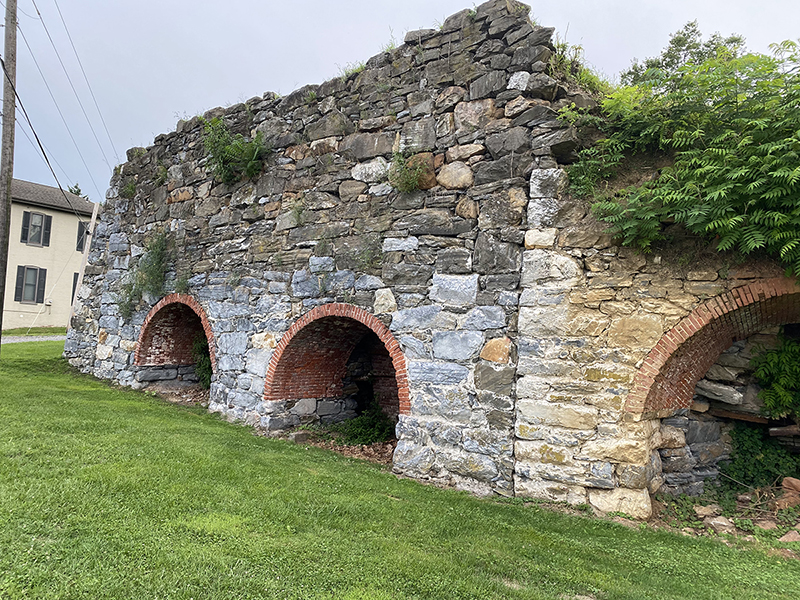The image depicts an old, broken-down stone structure resembling an abandoned irrigation system or old tunnel setup. Prominently in the foreground is a grassy area. The main cobblestone structure is centrally placed and made up of varying shades of gray, black, tan, and blue-ish stones. It features three distinct, semicircular archways, which are hollowed out and appear to serve an unclear purpose. As the wall extends to the right, the stones lighten in color, displaying hues of lighter blue and gray. At the top, the structure is overgrown with foliage, and there is evidence of another broken semicircular archway partially obscured by the greenery.

In the background to the left side of the image, there is a tan-brown building with brown windows and a brown roof, barely visible behind some vegetation. Additionally, an electric pole rises into the sky, though its top is out of frame. The scene is set under a clear, blue sky with a few clouds, and there are no people or text present in the image.